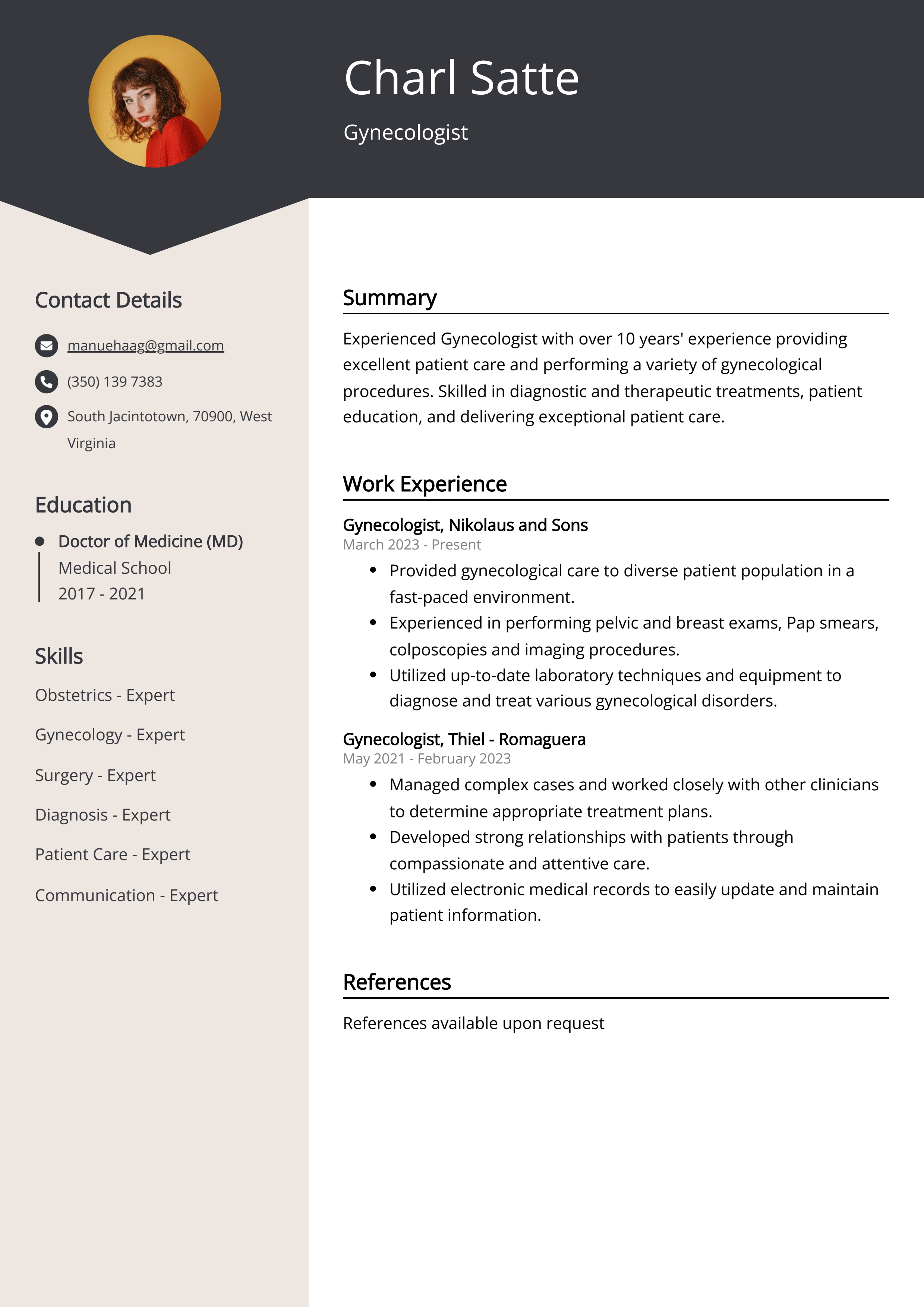The image is a detailed resume for Charls Satt, a gynecologist. Her name and occupation are prominently displayed in white letters against a very dark navy blue heading at the top. To the left, there is a photo of Charls Satt, a young woman with red shoulder-length hair, makeup, and a red sweater, set against a dark background. Contact details, including her email, phone number, and address, are placed below the picture within a large beige bar on the left side.

Charls has a Doctor of Medicine degree, obtained between 2017 and 2021, and possesses over 10 years of experience in the field of gynecology, providing excellent patient care and performing various gynecological procedures. Her skills include obstetrics, surgery, diagnosis, patient care, and communication. The resume also outlines her work experience from March 2023 to the present, where she has been managing complex cases and providing gynecological care to a diverse patient population. The resume concludes with a note that references are available upon request.